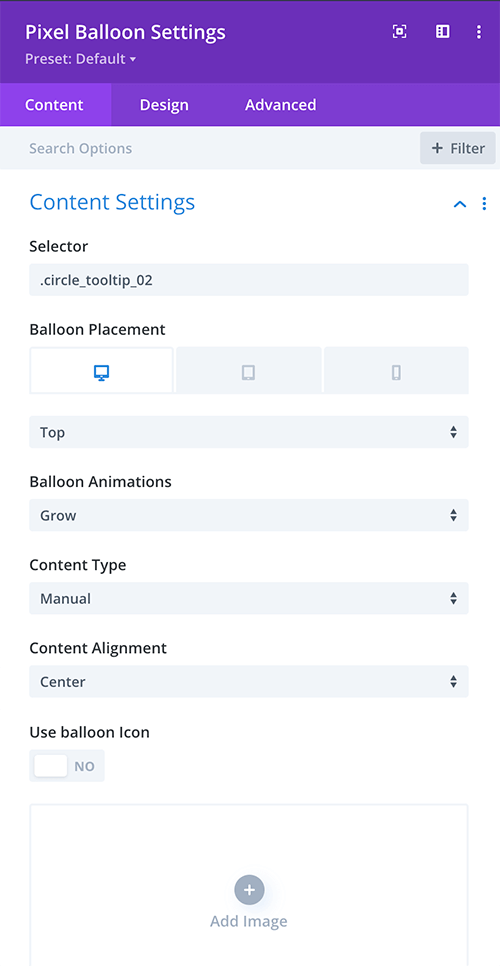This image likely showcases a screenshot from a mobile or tablet device, potentially a cropped desktop view, making the exact operating system indiscernible. Dominating the top part of the image is a purple background header with white text, bearing the title "Pixel Balloon Settings." The preset is currently configured to 'default.' To the right side of the header, there are icons representing a photo, a notebook, and a set of three vertical dots.

Beneath the header, there's a navigation menu in a lighter purple hue, with "Content" highlighted. Other options available in this menu include "Design" and "Advanced." A search filter is present, featuring a gray rectangle with a plus sign symbol.

The "Content Settings" section is expanded, revealing detailed configurations. The "Selector" is specified as ".circle_tooltip_02." For "Balloon Placement," users can choose between different device types, presumably desktop, tablet, or phone; currently, the option "Top" is selected from a dropdown menu. The "Balloon Animations" are set to "Grow," also from a dropdown menu. The "Content Type" is configured to "Manual," with alignment set to "Center," both controlled via dropdown menus. An option to "Use Balloon Icon" is toggled to 'No.' At the bottom of this section, there's an "Add Image" button marked with a plus sign.

This interface seems to be a configuration panel, possibly for a smart balloon feature, allowing users to customize how a pixel balloon appears and behaves across various devices.